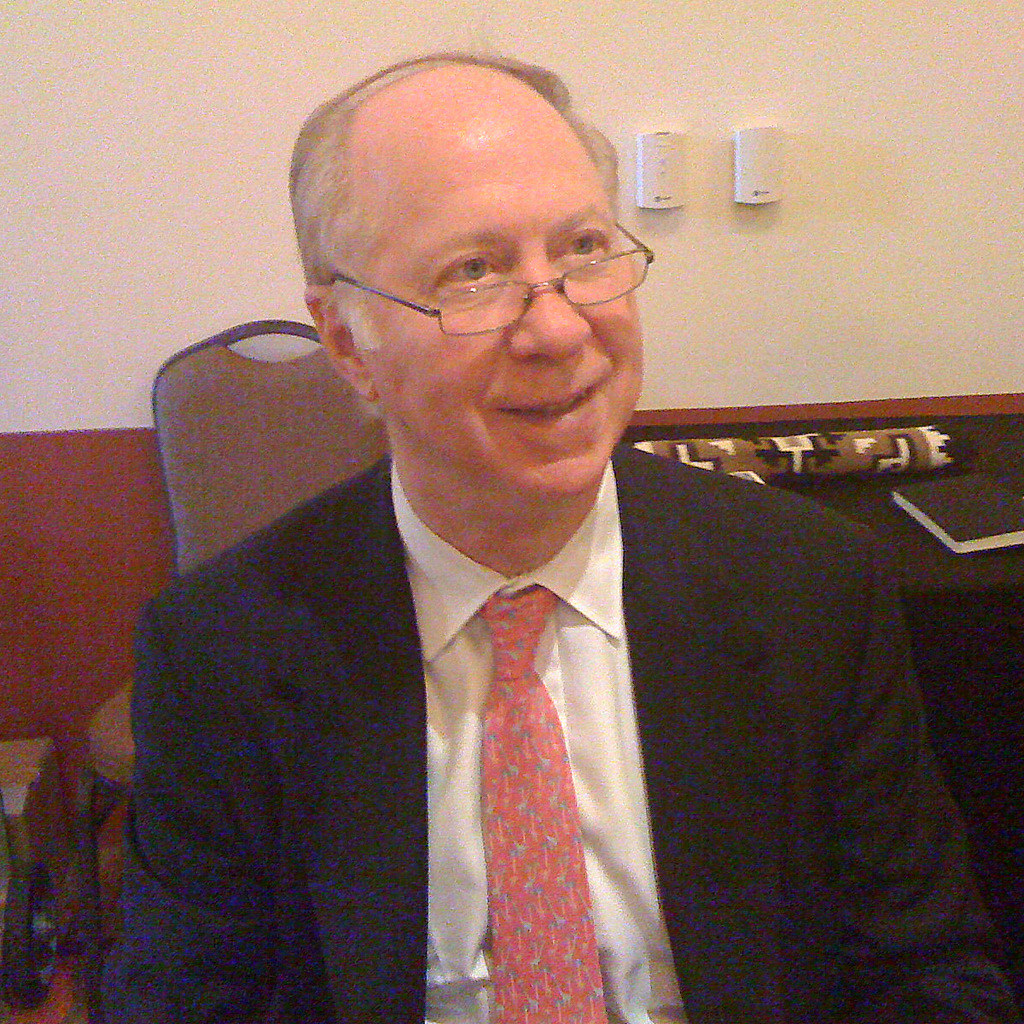The photograph captures an older, Caucasian man seated in a chair, visible from his stomach upwards, with the lower half obscured by the picture's edge. He is slightly hunched over, indicating he is sitting down. The man is dressed in a black business coat over a white button-up shirt, adorned with a distinctive pink tie featuring blue long-neck dinosaurs. His face, partially balding with a poorly done comb over, features silver hair on the sides and back of his head. Rectangular black-framed glasses rest on the bridge of his nose, through which his blue eyes are visible. He gazes slightly to the right of the frame, with his mouth open in a subtle smile that reveals the top part of his teeth.

In the background, to the left, a brown chair is visible while the wall behind him transitions from maroon at the bottom to beige at the top. On the right side of the frame, two plastic boxes, possibly AC control units, are mounted on the wall. Above his right shoulder, a woven material is rolled up on the table, accompanied by a black and white notebook, adding to the detailed setting of the image.